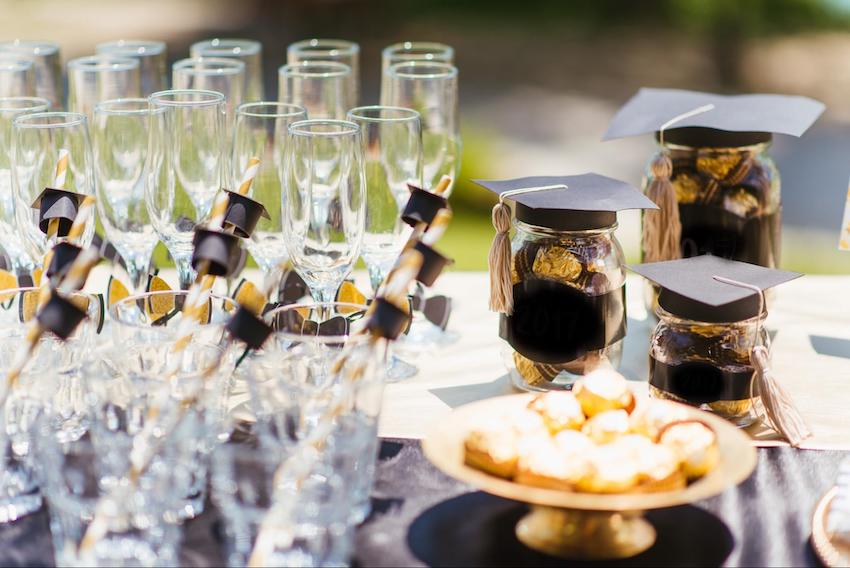The photograph captures a meticulously set-up table for a graduation party, adorned with a striking black and gold theme. Prominently, the table features several rows of clear wine stemmed glasses and tumbler glasses, each garnished with a swizzled stick or straw topped with a miniature black graduation hat. To the right, three mason jars filled with gold and black candies are capped with graduation hats, complete with tassels. In front of these jars sits a tray on a white plate with a gold base, holding what appear to be cookies or small cakes. The setting is completed with a black tablecloth, and the blurred background suggests a blend of green, blue, and brown hues. The entire arrangement conveys a festive yet sophisticated atmosphere, ready for the celebration.